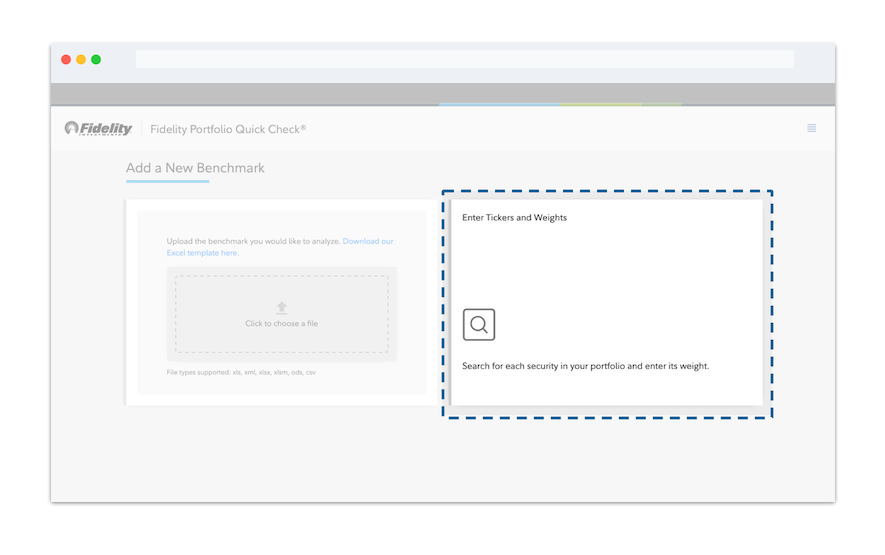In this detailed image of the Fidelity Investments interface, the focus is on the Fidelity Portfolio Quick Check page. The graphical user interface presents many familiar design elements associated with digital financial platforms. 

In the top left-hand corner, there are three small circles colored red, yellow, and green, mimicking traditional window control buttons. To the right of these circles is a rectangular search bar.

Following this, the page prominently displays the Fidelity logo next to the company's name. Immediately to the right in gray text, the title "Fidelity Portfolio Quick Check" is visible. Below this header, a slightly larger gray text invites users to "Add a New Benchmark."

The interface also features a functional section where users can interact with their benchmarks. This area includes a prompt that reads "Upload the Benchmark You Would Like to Analyze," followed by an option to "Download to Excel Template Here," suggesting that users can integrate Excel for their analysis.

To the right of this upload area, another interactive component allows users to enter specific financial information—a square-shaped search box prompting "Enter Tickers and Weights" followed by a clickable option to "Search for Each Security in Your Portfolio and Enter the Weight."

This interactive layout points to a comprehensive tool designed for detailed financial analysis and portfolio management.